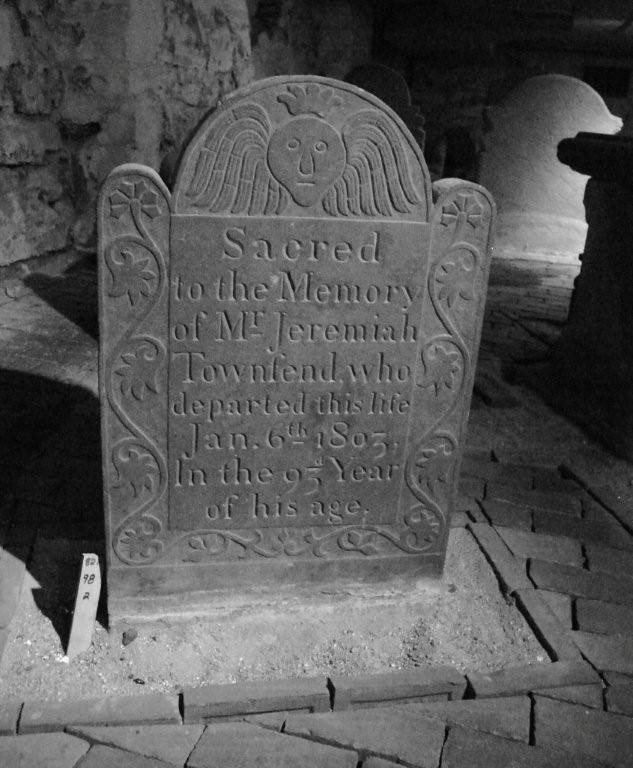This black-and-white photograph captures a detailed scene inside a mausoleum or similar structure. At the center, a small tombstone stands out, encased within a rectangular bordered area filled with sand, contrasting against the surrounding cobblestone floor. The tombstone bears intricate engravings; at the top, a half-circle arch frames a carved face with a long nose, angel wings, and a crown-like element. The inscription reads, "Sacred to the memory of Mr. Jeremiah Townfend who departed this life January 6, 1803 in the 93rd year of his age." Delicate engravings of flowers or vines adorn the borders of the headstone, enhancing its historical elegance. Next to the tombstone, a small marker is partially inserted in the sand, displaying the number '98.' The dimly lit interior reveals a stone-brick wall in the background, faintly visible due to the photograph's monochromatic scheme, creating an atmosphere of solemn reverence and timelessness.